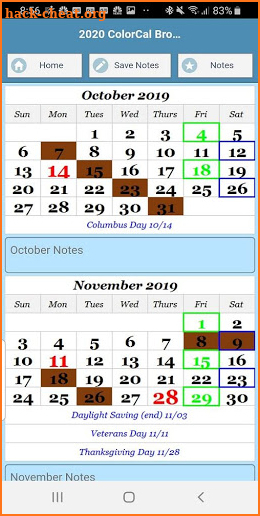The image shows a smartphone screenshot featuring a calendar from the website "back-cheat.org". At the top of the screen, various phone icons are visible, including the NBC logo, a time indication of 8:56, a muted microphone symbol, a battery life of 83%, and an active Bluetooth icon.

The main focus is a calendar displaying the months of October and November 2019, under the title "2020 ColorCal BRO...". This title is set within a blue box, with white formatting and follows three shortcut icons beneath it: "Home" (depicted with a house icon), "Save Notes" (represented by a pencil icon), and "Notes" (indicated with a star icon).

Below these shortcuts, October 2019 is displayed prominently in bold. The week headers run from Sunday through Saturday. On this calendar, notable highlights include:
- October 4th, highlighted with a green box
- October 7th, 15th, 23rd, and 31st, marked with brown boxes
- October 12th and 26th, outlined with a blue border
- October 14th, marked in red, with a note below indicating “Columbus Day 10/14"

Under October’s notes, there is a blank blue box. Moving on to November 2019, notable date markers are:
- November 1st, 15th, and 29th, highlighted with green boxes
- November 8th, 9th, 18th, and 26th, marked with brown boxes
- November 9th and 23rd, outlined with a blue border
- November 11th and 28th, with dates marked in red

Important dates noted below include:
- “Daylight Savings Ends 11/03”
- “Veterans Day 11/11”
- “Thanksgiving Day 11/28”

Finally, there is a blue box labeled “November Notes” which is currently blank.